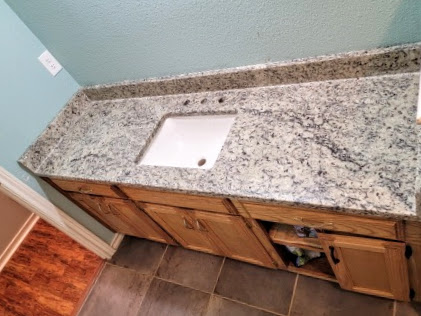This image captures an in-progress bathroom renovation, showcasing a sink vanity area. The floor features a tile pattern in shades of gray and white, with off-white grout. Adjacent to the bathroom, the floor transitions to a reddish-brown wooden finish. The vanity wall is painted in a soft pale blue color, complementing the gray and white marble countertop. The countertop includes a large, white sink basin with a visible drain hole, yet it lacks the faucet and handles designated for hot and cold water, suggesting that installation is incomplete.

Spanning the width of the countertop, the ample space could potentially accommodate additional sinks, conducive to a dual or triple basin setup if plumbing permits. Below the countertop, wooden cabinetry is evident. The facade includes what appears to be three decorative drawer fronts, though only one drawer is functional and accessible. Additionally, there are three sets of wooden cabinets, each equipped with vertically oriented silver handles. Two of these cabinets are closed, while the third is missing its left door. The remaining right door hangs precariously, indicating it may also detach soon. Within the open cabinet, some items are visible but indistinguishable, highlighting the space's unfinished state.

Overall, this image depicts an incomplete bathroom setup, with a partially installed sink and cabinetry awaiting further assembly.